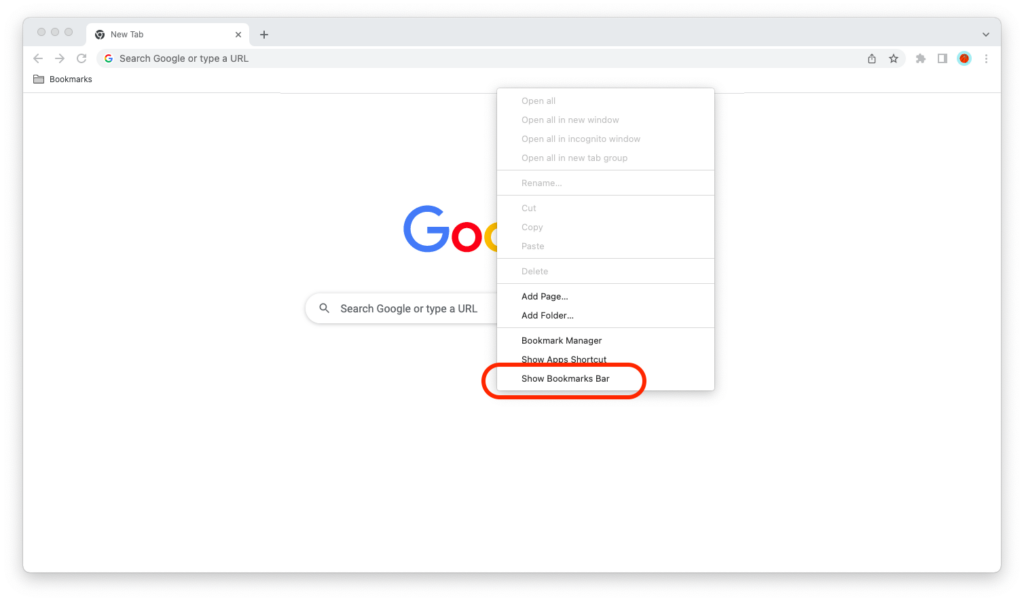The image depicts an open browser window featuring the various icons and user interface elements typically found in a web browser. At the top, there is a file tab bar with clickable options for new tabs and navigation arrows. To the right of these, a refresh button sits alongside a "G" icon, indicative of a Google search bar or branded feature. The search bar itself is receiving focus, implying it is active, suggesting the user can type a URL or search query. Beside it are multiple icons: a square arrow, a hollowed-out star for bookmarking, a puzzle piece for extensions, and additional settings circles.

Below, a dropdown menu appears, offering actions such as "open all," "open in new window," "open in new tab group," and further management options like rename, cut, copy, paste, delete, add page, add folder, and access the bookmark manager. These actions are visually represented with red and gray ovals and text options. The shadowy gray top edges imply a layered window view or a focused modal providing these options.

The underlying theme seems to involve bookmarks and browser management, as indicated by commands to show and organize bookmarks. Additionally, the area with the red oval showcases the text "show bookmarks bar," suggesting enhanced functionalities for user convenience. The subtle shadow effects combined with the color-coded icons create a structured and intuitive user interface, typical of modern web browsers.